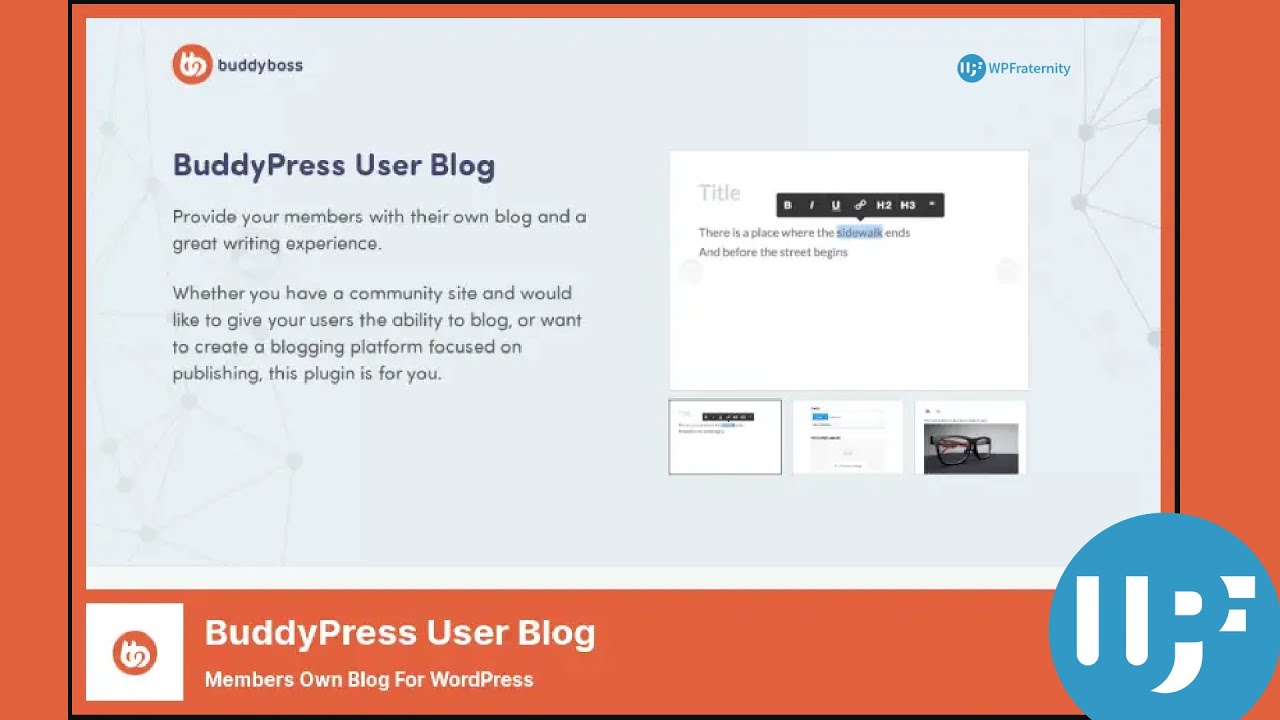In the center of the image, there is an orange-bordered square with various design elements and text. At the bottom of the square, a white box contains the text "BuddyPress User Blog" in white lettering. Below this, smaller text reads, "Members own blog for WordPress." To the far right, a blue circle is present with two white vertical lines inside and a white semicolon next to it.

At the top of the square, "BuddyBoss" is written with an orange circle beside it. Below this, the text "BuddyPress User Blog: Provide your members with their own blog and a great writing experience" is displayed. The next paragraph reads, "Whether you have a community site and would like to give your users the ability to blog or want to create a blogging platform focused on publishing, this plugin is for you."

To the right inside the square, there is a text block with the phrase "There is a place where the" followed by the word "sidewalk ends" highlighted in blue, continuing with "and before the street begins." In the very bottom right corner, there is an image of black-framed eyeglasses resting on a black table, set against a gray background.